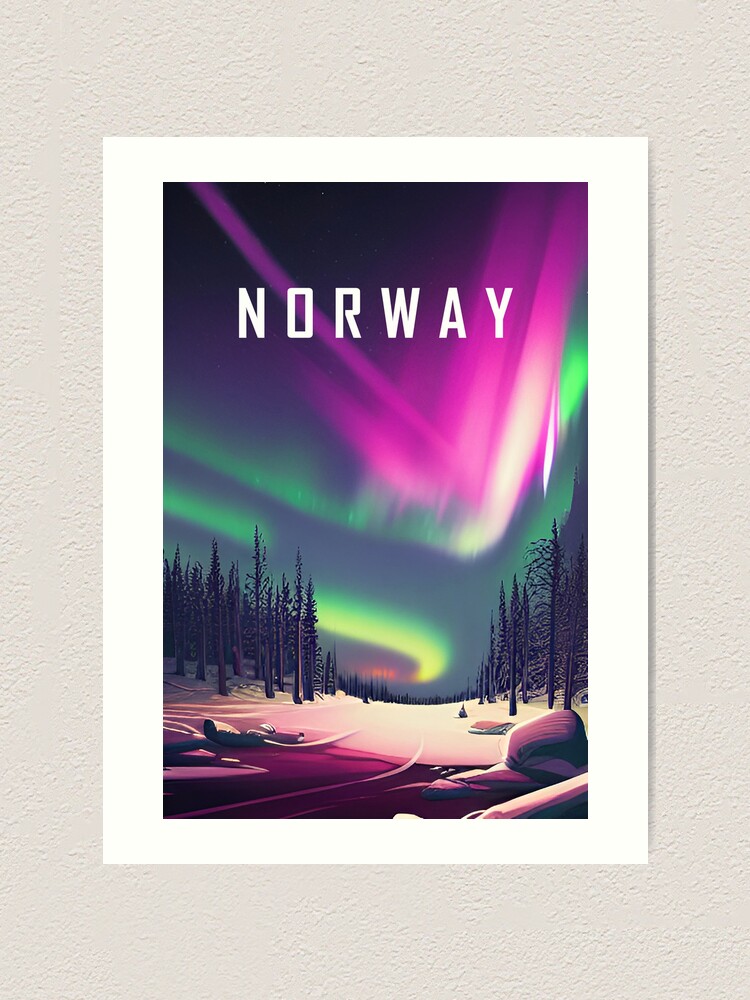This photo showcases a beautifully stylized poster advertising Norway, prominently displayed on a beige wall. The poster, framed and matted with a gray and white double mat, features a striking central image bordered by white. Captured at night, the scene highlights the awe-inspiring Northern Lights, with swirls of green, blue, deep purple, pink, yellow, and orange dancing across the sky.

Below the luminous aurora, a snow-covered landscape stretches across the bottom, dotted with rocks and boulders. A stark, open space resembling a road cuts through the center, flanked by tall pine trees on either side. In the middle of the radiant lights, the word "Norway" stands out in bold, white font, adding to the poster's visual appeal. The deep purple hues near the bottom transition seamlessly into a vibrant display of colors, making the poster both eye-catching and evocative of Norway’s natural beauty.